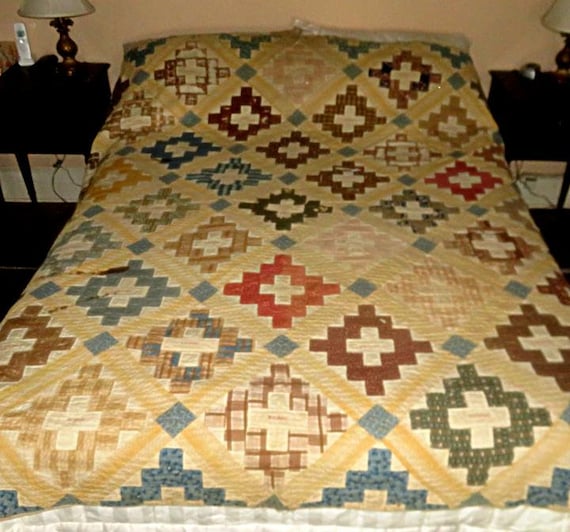The photograph depicts a vintage or retro-styled bedroom, with a prominent bed covered by a lively, multicolored quilt. The bed is flanked by two nightstands, each adorned with matching lamps featuring dark brown bases and white shades. A detail of a house phone on the left nightstand enhances the period feel. The quilt, which is the centerpiece of the image, showcases a dominant yellow hue with a dynamic pattern of stepped diagonal squares. These squares create a staircase effect from corner to corner, intersected by yellow X's that converge with blue diamonds. This intricate patchwork also includes a variety of colors, such as blue, green, red, brown, and pink, forming small pixelated diamond shapes within each square. The room's walls are a light peach color, complemented by a white border at the bottom, adding to the nostalgic ambiance of the scene.